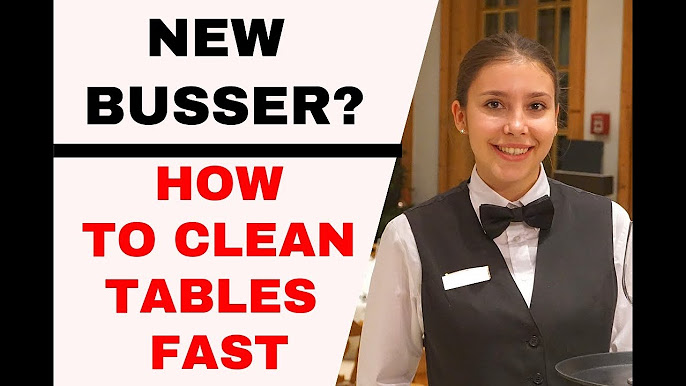The image appears to be part of an informational tutorial, likely a screenshot from a video or PowerPoint presentation aimed at new bussers. The image is bordered by vertical black areas on both the left and right sides. At the top left, bold black capital letters spell out "NEW BUSSER?" followed by a horizontal black line. Below this line, in large red capital letters, the text reads "HOW TO CLEAN TABLES FAST."

On the right side of the image, a young girl or teenage girl is featured. She has a slightly tanned complexion, brown eyes, and black hair pulled back into a ponytail. She is smiling and wearing small earrings, a white long-sleeved button-up shirt, a black vest, and a black bow tie. She appears to be a waitress or busser, holding a tray as if ready to serve food or drinks. Behind her, there is a door and a fire alarm, as well as some tables, indicating a restaurant setting. The overall aim of the image seems to be to provide tips or instructions on efficient table cleaning for new bussers.